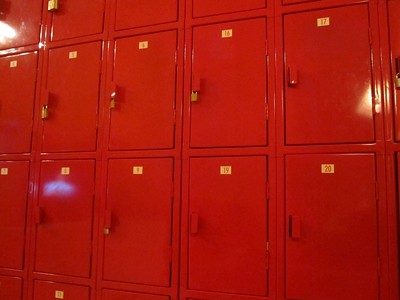The image displays a close-up of cherry red metal lockers, possibly from a gym, swimming pool, or high school hallway. The lockers, which are small in size, are arranged in at least four visible rows with each locker featuring a white tag bearing red numbers within a gold box. Visible numbers include 13 through 17 on the upper rows and extend to 20 in the bottom rows, though the exact grouping of the lockers is ambiguous due to cut-off edges. Some lockers are secured with uniform gold padlocks, while others remain unlocked. The image captures a slight blue glow on one of the lockers near the bottom and reflects a sheen from the light source located at the top left, resulting in a glare on several lockers, particularly in the top left corner. The photo is taken from a low angle looking upward, contributing to its somewhat unclear and incomplete view.